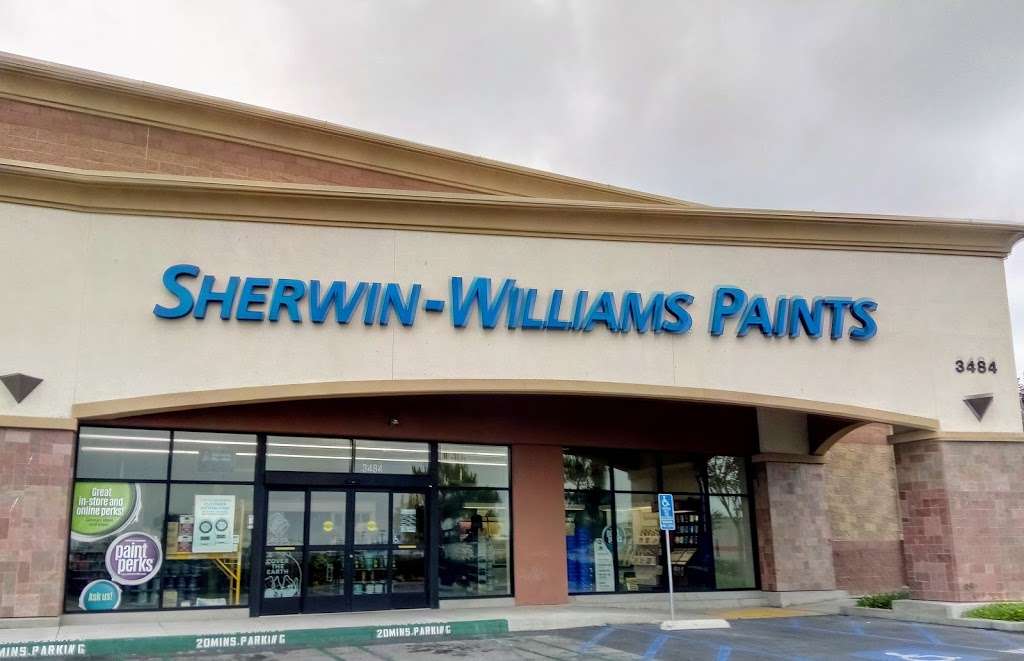The photograph depicts the front facade of a Sherwin-Williams paint store. The building features a beige cement upper section that prominently displays the "Sherwin-Williams Paints" sign in bold blue letters. Below, the structure transitions into a brownish brick facade. Centrally located under the sign are the main entrance doors, consisting of four glass doors. To the left of these doors, several promotional signs are visible, likely advertising sales or special offers. The right-hand side of the building's front wall displays the address "3484" in clear numbers. Extending from the building is a parking lot, which includes designated wheelchair-accessible parking spaces, though it is currently devoid of vehicles.